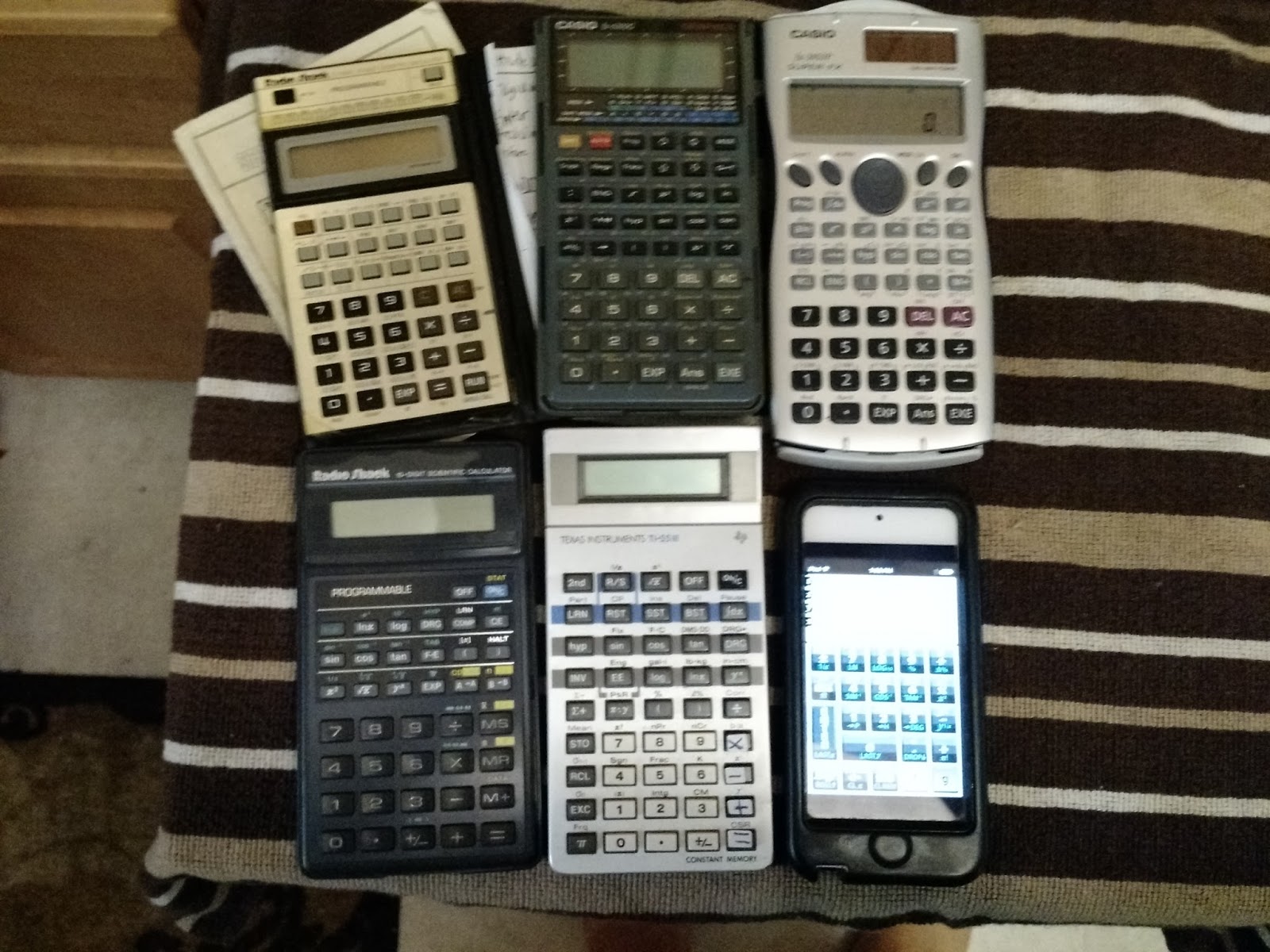The image features six old-school calculators resting on a slightly blurry, horizontally striped cloth with various shades of dark brown, white, and light brown. Arranged in two rows of three, the calculators showcase a mix of vintages and brands, including RadioShack and Casio models. The top row includes a silver calculator, a black calculator, and another silver calculator, while the bottom row has a black calculator, a white calculator, and a device resembling a cell phone with touch buttons. Some of the calculators have red keys, and a couple are turned on, displaying digital readouts. Behind the calculators, there are pieces of paper, possibly receipts or notes. The cloth is striped in dark brown, white, and tan, forming a subtle backdrop. The overall composition appears casual, perhaps for documentation or sale.